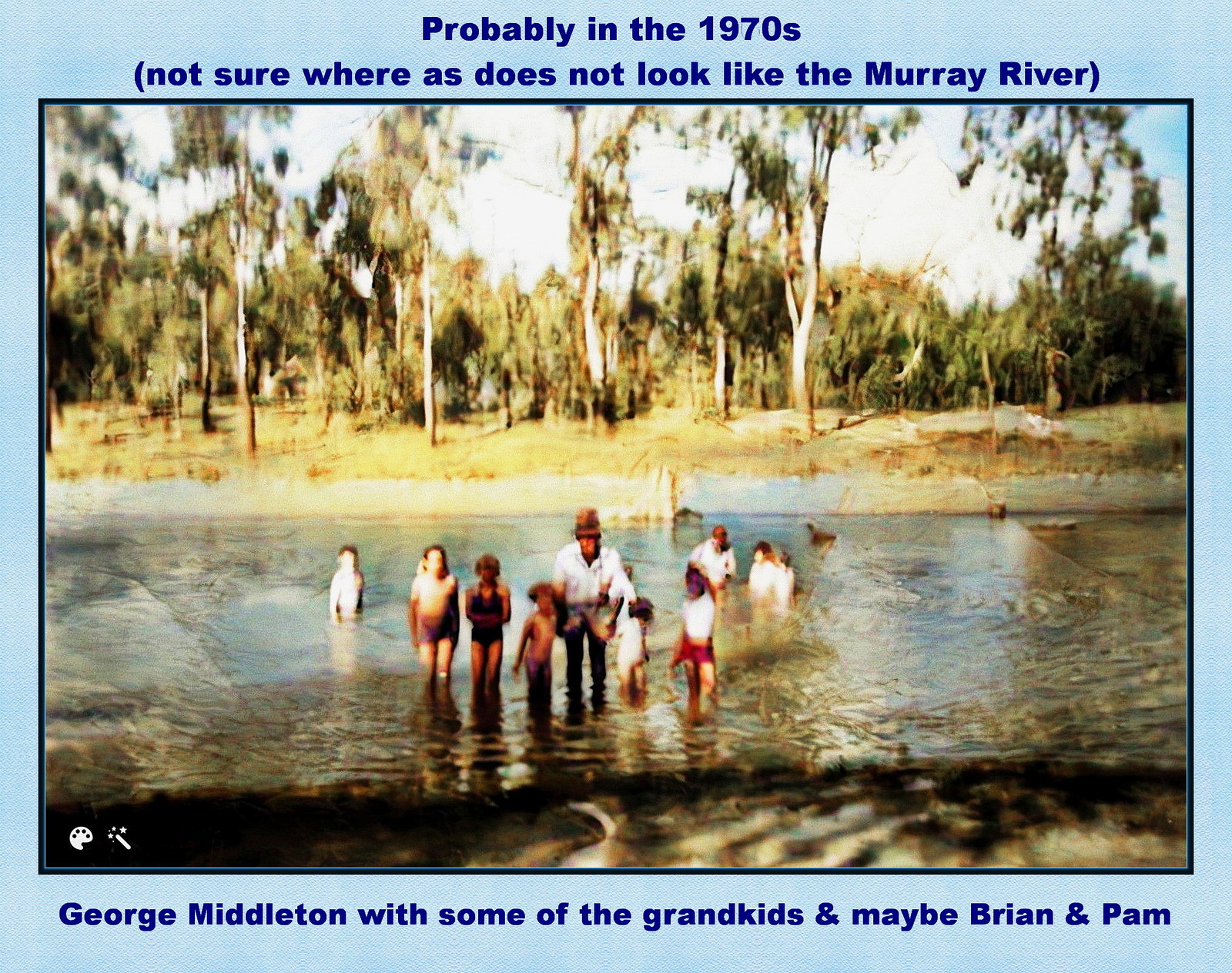The slightly blurry, color photograph, inset within a teal-colored box with dark blue text, captures a sunlit, outdoor scene likely from the 1970s, though its precise location is uncertain as it "does not look like the Murray River," according to the caption. The image features a black man, identified as George Middleton, wearing a white button-down shirt, dark shorts, and a wide-brimmed, brown fedora reminiscent of Indiana Jones. He stands in the middle of a river or lake, surrounded by a group of at least eight children and possibly a couple of adults in the background. Some children, dressed in bathing suits, have varying skin tones, which might be influenced by the sunlight. The waterway stretches from left to right, with a grassy shore and tall trees with high canopies in the background, creating a serene natural setting. The text below the photo mentions the man as "George Middleton with some of the grandkids and maybe Brian and Pam."